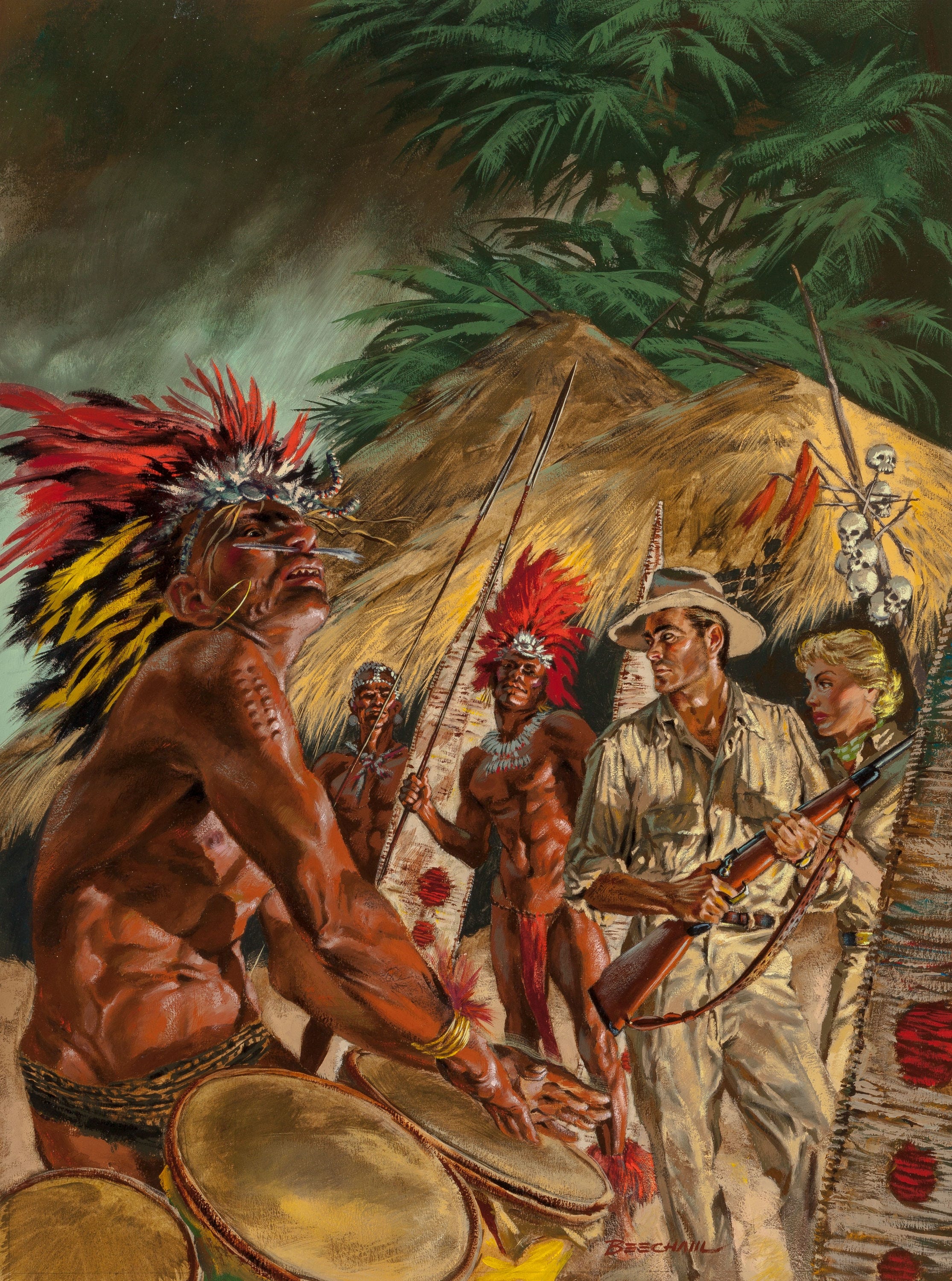The painting depicts a striking scene set in a tropical land during an earlier time period. Dominating the composition is a muscular Indigenous man with a feathered headdress in hues of red, yellow, and white, along with a piercing through the skin between his nostrils. He is positioned slightly to the left, facing the viewer while playing a set of three drums. He is adorned in a loincloth and appears deeply engrossed in his music. Standing behind him are two fellow tribesmen, similarly dressed in red loincloths and shell necklaces, holding long spears.

In the background, the landscape is rich with green, leafy palm trees and thatched huts crafted from yellow and brown materials. The sky looms dark and ominous, transitioning to a lighter shade near the horizon. To the right, two Caucasian figures stand facing the drummer. The man, dressed in tan safari attire reminiscent of Indiana Jones, holds a rifle across his body. The blonde woman beside him, also in tan clothing with a green scarf, glances off to the right, her hair pulled back into a bun. Notably, a pole adorned with skulls and red ribbons stands amongst the huts, adding to the scene's exotic and historical atmosphere. At the bottom middle of the painting, the artist's signature, "Beach Hail," is clearly visible.